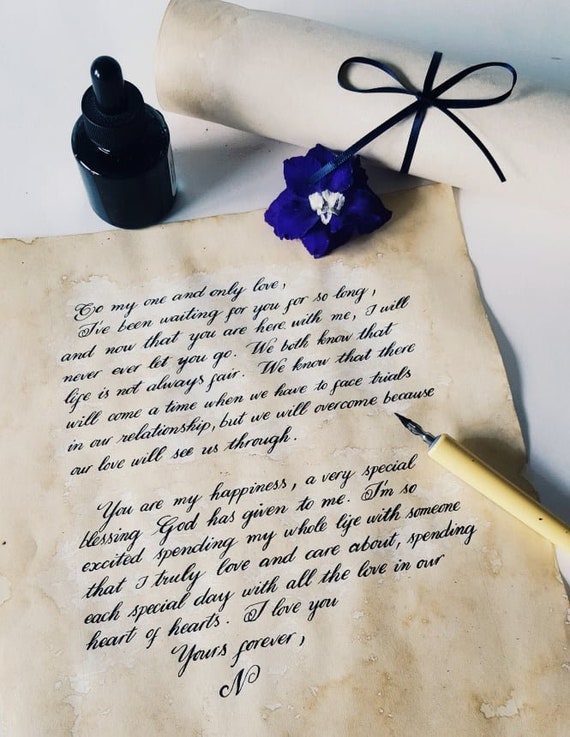In the detailed image, there is a close-up of a letter written on aged, faded parchment paper, featuring dark spots that add to its vintage appearance. The letter is penned in elegant cursive using a quill ink pen, with the ink holder placed adjacent to the parchment. To the right of the letter is the ink capsule, used to dip the pen for writing.

The parchment bears a heartfelt message: "To my one and only love, I've been waiting for you for so long and now that you are here with me, I will never let you go. We both know that life is not fair. We know that there will come a time when we have to face trials in our relationship, but we will overcome because our love will see us through. You are my happiness, a very special blessing God has given to me. I'm so excited spending my whole life with someone that I truly love and care about, spending each special day with all the love in our heart of hearts. I love you, yours forever in."

In the upper-left corner of the image, there is a rolled-up scroll tied with a thin black ribbon, accentuating the historical feel. A delicate blue flower is attached to the parchment, adding a touch of decorative elegance. The entire composition appears to be an evocative recreation of 17th-century correspondence, perfectly capturing the romantic and timeless essence of the period.